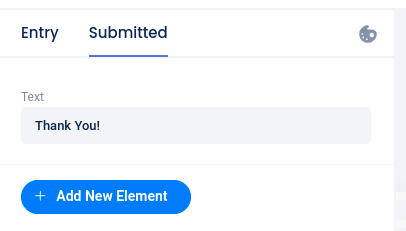The image showcases a digital interface, likely from a mobile device or tablet, featuring a structured layout with distinct sections. At the top of the screen, there's a gray bar containing text, though the specific content is unclear. Below, two prominent black-labeled tabs read "Entry" and "Submitted," indicating different stages or categories within the application. Another noticeable section includes the word "Text" in black font, and directly underneath, a gray bar that appears to be a text input area.

There's a blue tab bar at the bottom of the screen with white lettering, highlighted by the phrase "Add New Element," inviting user interaction. The term "Thank you" is displayed in black text within the interface, possibly as a form of acknowledgment or confirmation message. At the top right corner, a small icon resembling a painter's palette is visible, suggesting an artistic or creative tool might be part of the application's functionality.

The overall color scheme is minimalistic, featuring primarily white, blue, gray, and black elements. The interface lacks additional visible context, such as device type or platform, leaving it ambiguous whether it's being viewed on a phone, tablet, or potentially a small segment of a larger screen.